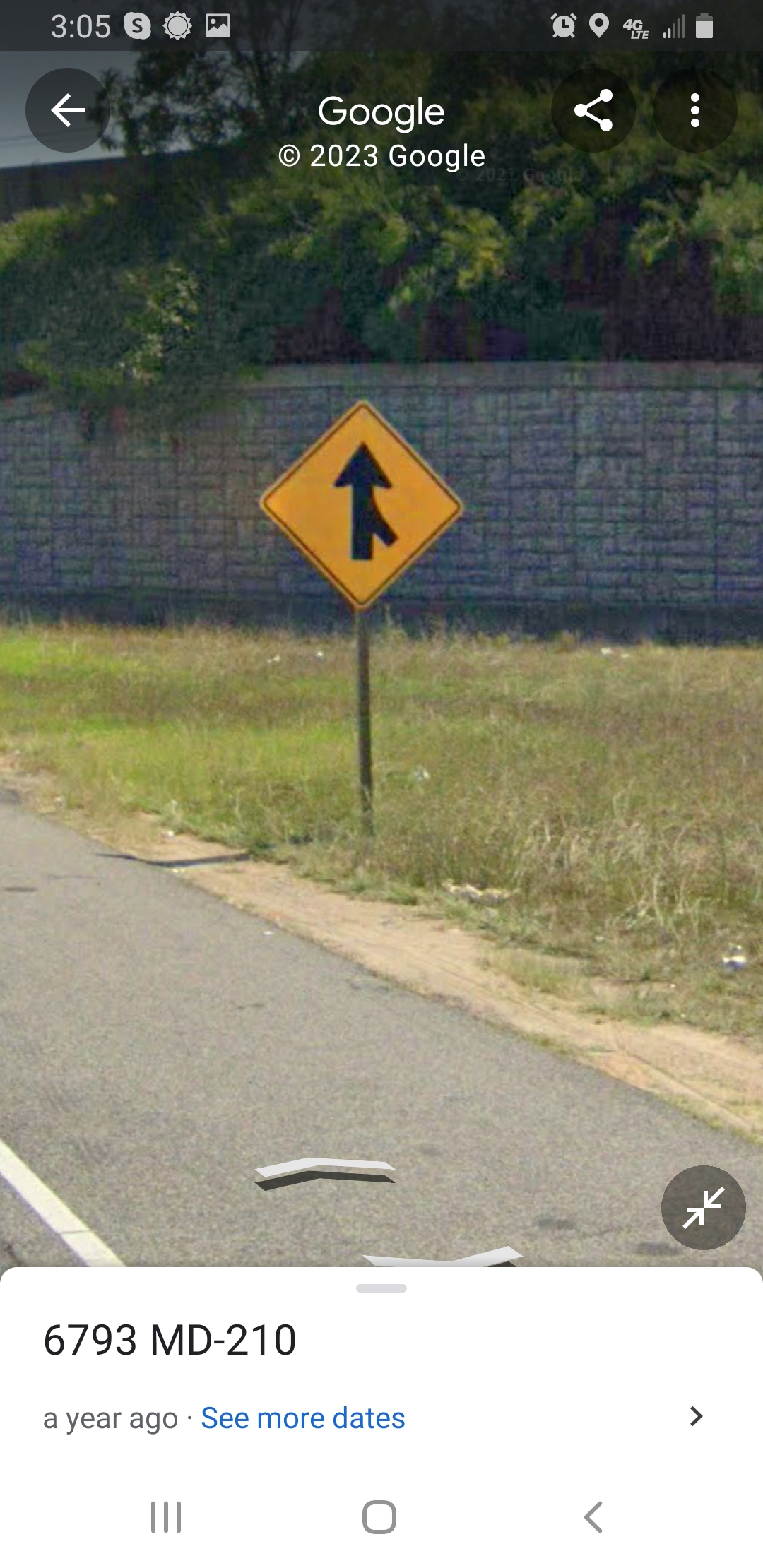The image is a screenshot captured from a cell phone, displaying a Google Maps view dated 2023. The focal point of the image is a yellow diamond-shaped street sign with a black merging arrow, indicating an upcoming merge. The sign is mounted on a rusted metal pole, standing in slightly overgrown grass. The scene features a gray brick retaining wall or sound barrier running parallel to the roadway. Directly behind the wall, several large, leafy green trees mark the season. Part of a highway is visible in the foreground, specifically the white line demarcating the extreme right-hand side of the right-hand lane, suggesting this could be near an on-ramp or off-ramp. The smartphone's overlay includes various icons: the time (305), weather, a clock, a location pinpoint, and a 4G LTE indicator. Just above the bottom of the screenshot, black text reads "6793 MD 210," with additional interface icons for navigation and settings. The scene encapsulates a typical day in a suburban or semi-urban setting, conveying both the technological and natural elements present.